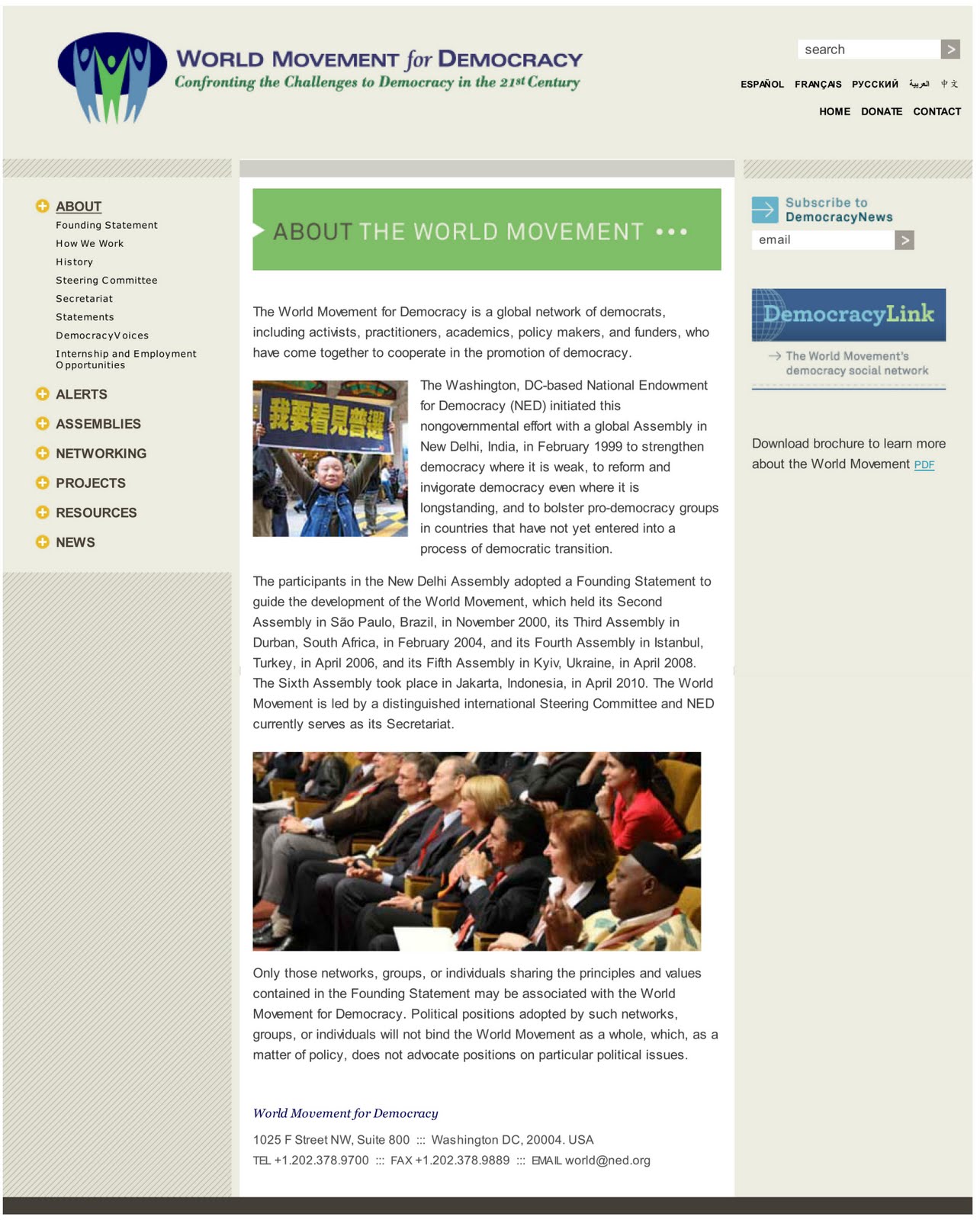The image features a banner at the top with text written in blue and green: "Wild Movement for Democrats, Confronting the Challenge to Democracy in the 21st Century." Below the banner, there is an illustration of three people holding hands. The central figure is green, and the two figures flanking either side are blue.

In the top right corner, there are interactive elements including a search box, language selection options, and navigational links labeled "Home," "Donate," and "Contact." A side menu on the left lists various sections: "About," "Funding Statement," "How We Work," "History," "Steering Committee," "Secretariat," "Statement," "Democracy Voices," "Internship and Employment Opportunities," "Alert," "Assemblies," "Networking," "Projects," "Resources," and "News."

The central portion of the page features a headline "About the Wild Movement," followed by an article detailing the organization's mission and history. The article states that the Wild Movement for Democracy is a global network comprising democracy activists, practitioners, academics, policymakers, and funders. Initiated by the Washington D.C.-based National Endowment for Democracy (NED) with its first global assembly in New Delhi in February 1999, the movement aims to strengthen fragile democracies, reform and invigorate longstanding ones, and support pro-democracy groups in undemocratic nations. Subsequent assemblies took place in São Paulo, Brazil (November 2000), Durban, South Africa (February 2004), Istanbul, Turkey (April 2006), Kiev, Ukraine (April 2008), and Jakarta, Indonesia (April 2010).

The Wild Movement is overseen by an international steering committee and currently has NED serving as its secretariat. Only network groups and individuals adhering to the principles and values in the funding statement may associate with the Wild Movement. As a policy, the coalition does not advocate for particular political positions; member groups and individuals are individually responsible for their political stances.